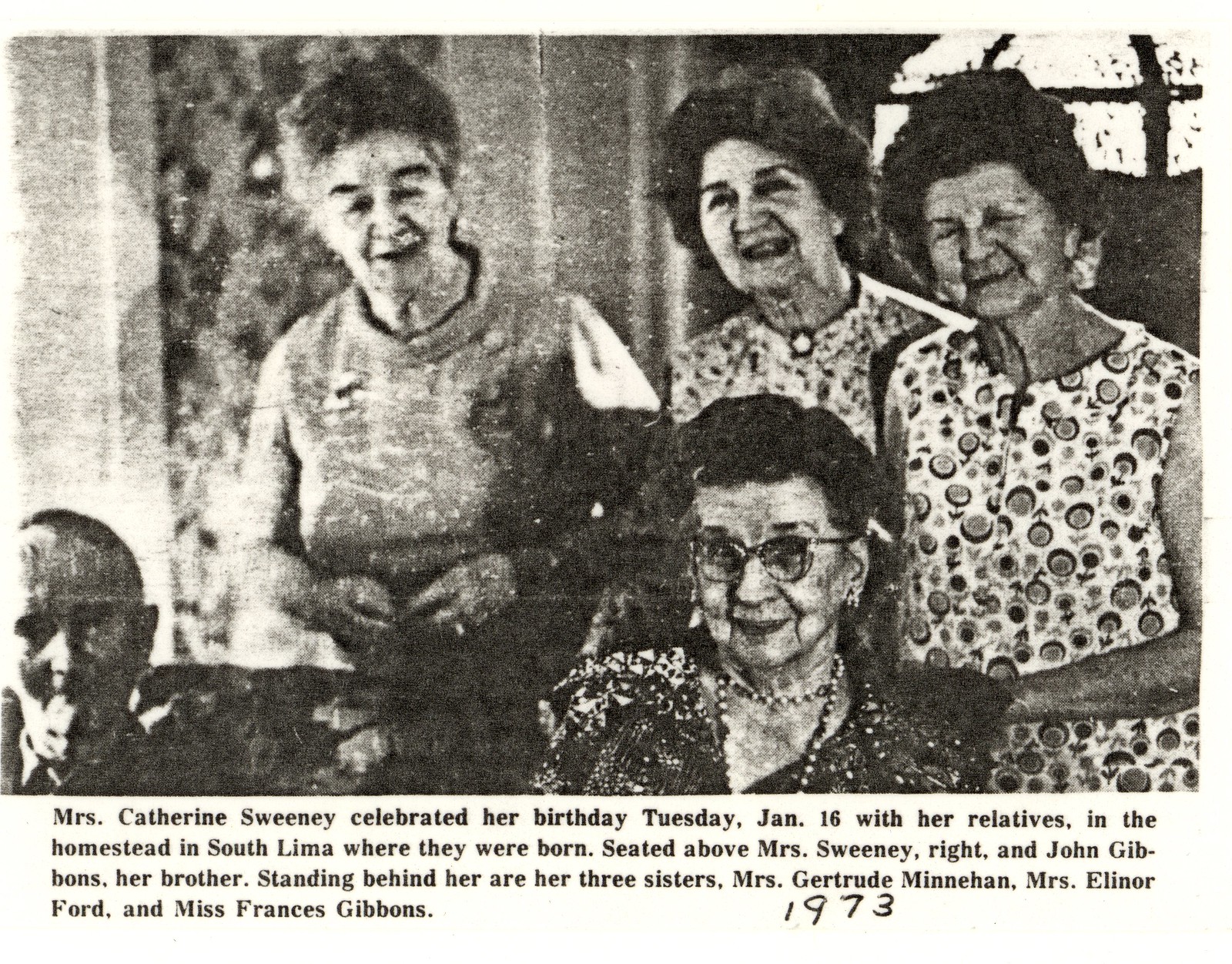The black-and-white photograph is a grainy image of five elderly individuals, four women and one man, gathered together to celebrate a special occasion. The women, all with short, permed black or brown hair and wearing dresses, are positioned around a seated woman adorned with pearls and glasses. Three of them stand behind her, while one woman is seated next to an elderly man in the bottom left corner. The setting appears to be inside a home in South Lima, featuring a window at the top right and what looks to be drapes on the left. Beneath the image, a caption reads, "Ms. Katherine Sweeney celebrated her birthday Tuesday, January 16 with her relatives in the homestead of South Lima where they were born." It further identifies the individuals: seated beside Ms. Sweeney is her brother, John Gilbons; standing behind her are her three sisters, Mrs. Gertrude Minahan, Mrs. Eleanor Ford, and Ms. Frances Gibbons. The year "1973" is handwritten below the printed text.